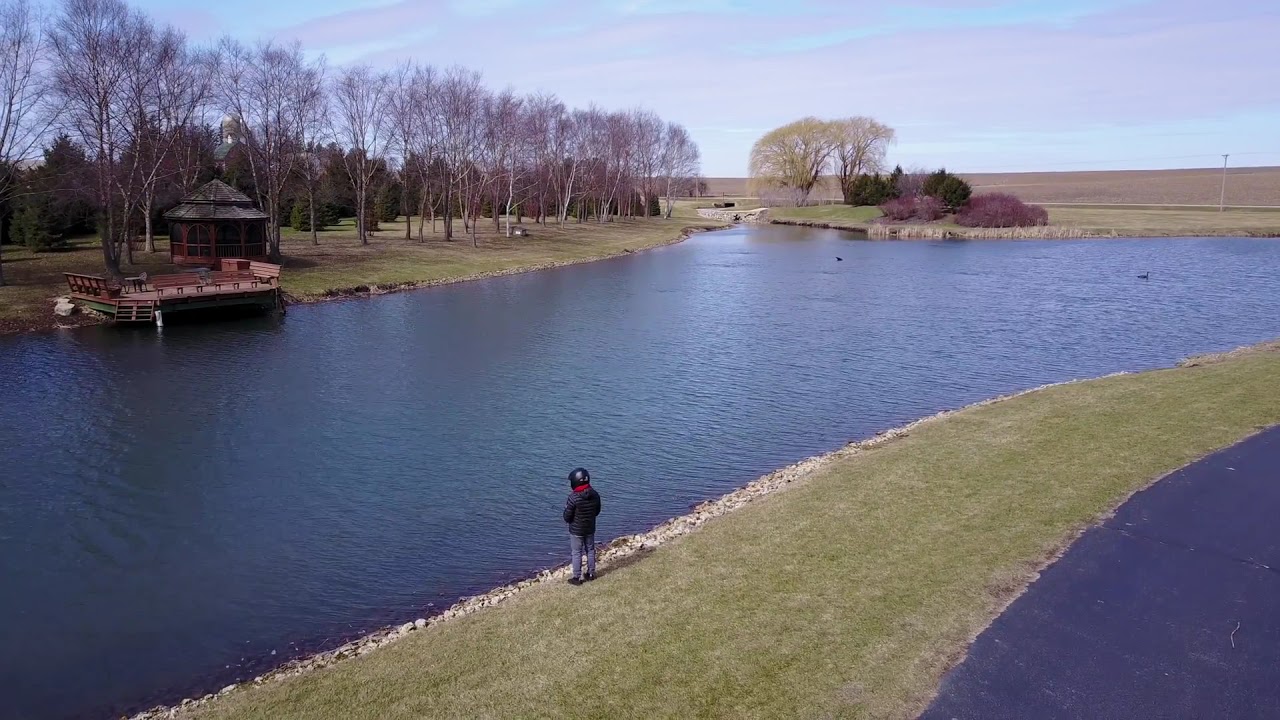This is a detailed photograph of a serene park landscape featuring a calm, blue water body, possibly a pond or a small lake, taken from an elevated vantage point. The water body lies centrally in the image, extending outwards towards both the left and right. On the right shore, a person, possibly a little boy based on one description, is seen standing on a green patch of grass. He is wearing a black helmet, black jacket, and blue jeans, and is looking into the water. He appears to be holding a black fishing pole and stands near a gravel path but is not on it. The shoreline around him is lush with green grass.

On the left shore, there is a wooden structure described variably as a gazebo or a boat dock, accompanied by an overlook deck extending to the water's edge. This area is dotted with trees, some of which are bare while others have leaves, and the ground shows a mix of greenery and brown patches. The sky above is a clear blue with some clouds, suggesting a crisp, potentially cold day. The overall scene appears natural and peaceful, depicting a typical park setting.